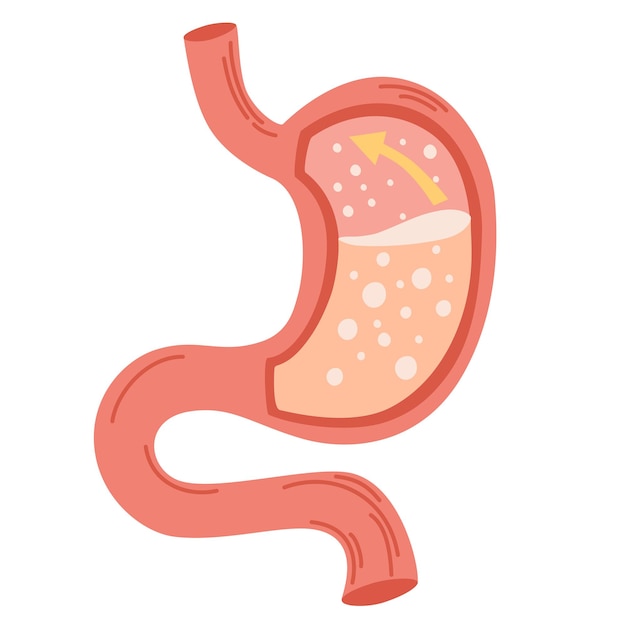The image depicts a detailed and colorful illustration of an anatomical organ, which could be interpreted as either a stomach or a kidney, placed against a stark white background. The organ is predominantly a bright, salmon pink color with connected tubes, signifying entry and exit points. Inside the organ, there is a beige-colored liquid, interspersed with numerous white circles representing air bubbles. A prominent yellow arrow, situated in the upper part of the organ, points upwards towards the gastrointestinal tubes, indicating the direction of fluid or gas movement. The fluid in the organ appears to be halfway filling it, and the bubbles are distributed from the bottom to the top of the internal cavity. Notably, the image contains no textual labels, leaving the viewer to rely solely on visual information, suggesting its use in an educational context such as a textbook illustration.